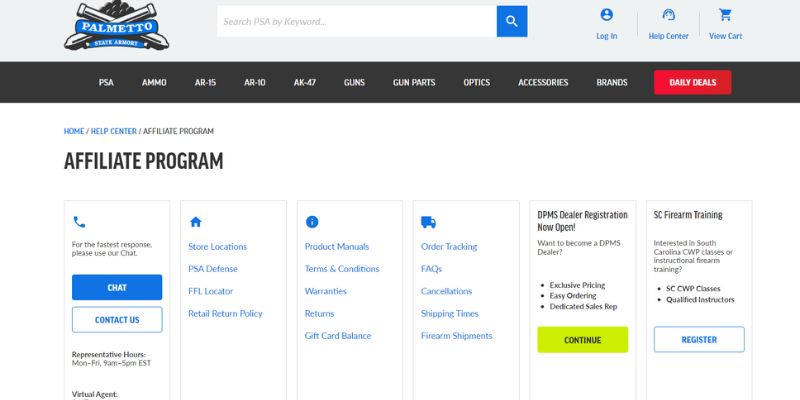The image depicts the homepage of the Palmetto State Armory website. At the top of the page, there's a prominent search bar labeled "Search Palmetto State Armory by keyword," alongside buttons for Login, Help Center, and View Cart.

Below, there is a navigation bar with clickable sections titled: PSA, Ammo, AR-15, AR-10, AK-47, Guns, Gun Parts, Optics, Accessories, Brands, and Daily Deals. The user navigated through several sections including Home, Help Center, and Affiliate Program.

Further down, multiple informational boxes provide contact options and important details. For quick assistance, there’s a chat feature with representative hours listed as Monday through Friday, 9 a.m. to 5 p.m. EST. Other informational boxes highlight Store Locations, PSA Defense, FFL Locator, Retail Return Policy, Product Manuals, Terms and Conditions, Warranties, Returns, Gift Card Balance, Order Tracking, FAQs, Cancellations, Shipping Times, and Firearm Shipments.

Additionally, there's a highlighted announcement about the DPMS Dealer Registration being open, encouraging users to become DPMS dealers for exclusive pricing, easy ordering, and access to a dedicated sales representative. Another box promotes South Carolina firearm training, inviting users to register for CWP classes or instructional firearm training sessions.